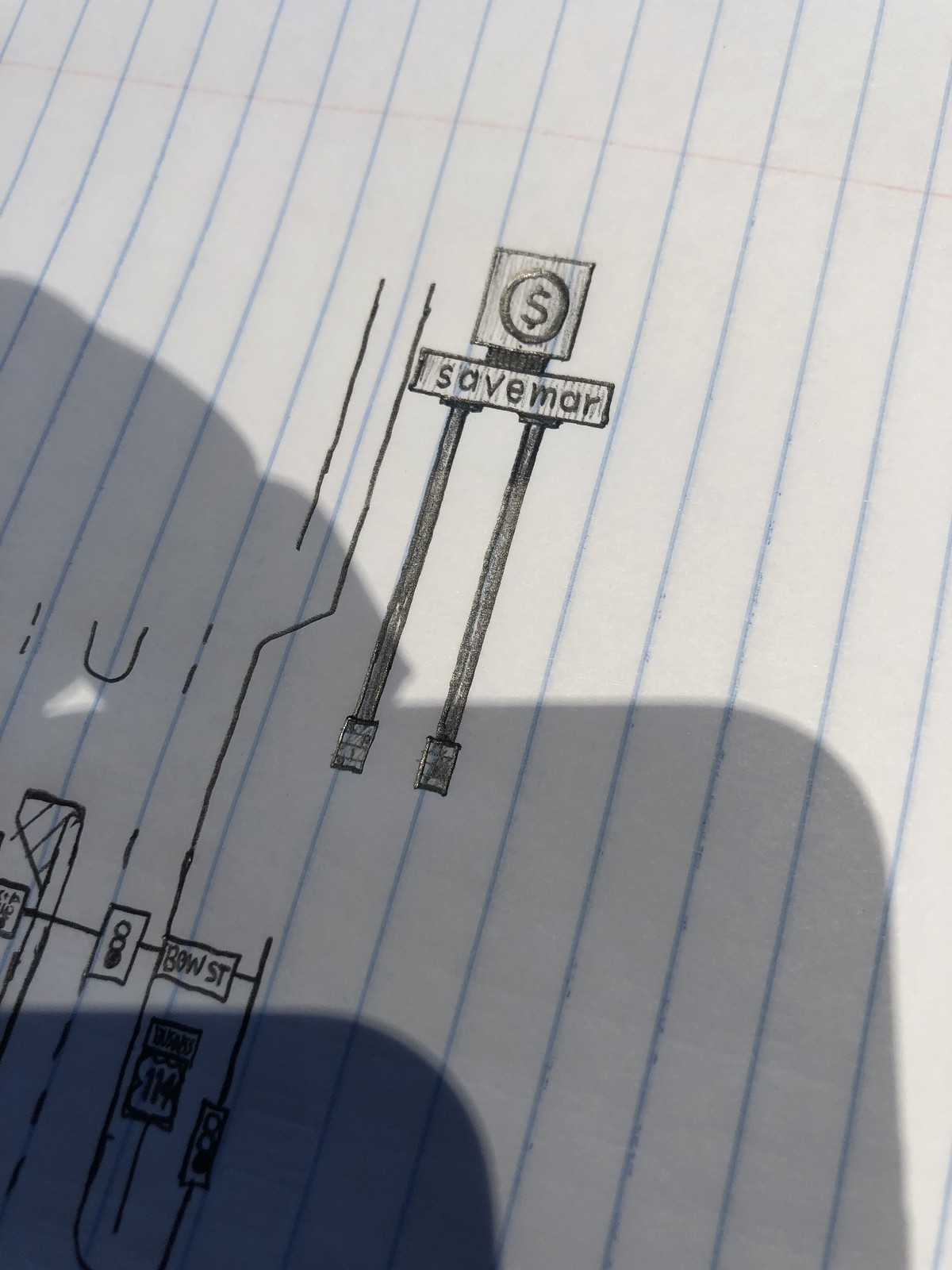In this photo, we see a detailed hand-drawn sketch on college-ruled white paper, characterized by its blue lines. The drawing appears to be a part of an accident reconstruction or street layout description. Dominating the center of the sketch is a billboard, prominently inscribed with the words "Save Mar." Above this text, there is a simple logo, a circle with a dollar sign at its center, both depicted in silver. The billboard is upheld by silver-colored poles that seem to be anchored into the ground with supporting cement or brick beams. To the side, there is an incomplete but recognizable drawing of a street, showing a few lanes. At the bottom of the drawing, traffic lights are illustrated, enhancing the depiction's realism. Additionally, a small sign with the label "Bow Street" suggests the specific intersection being represented in the scene.